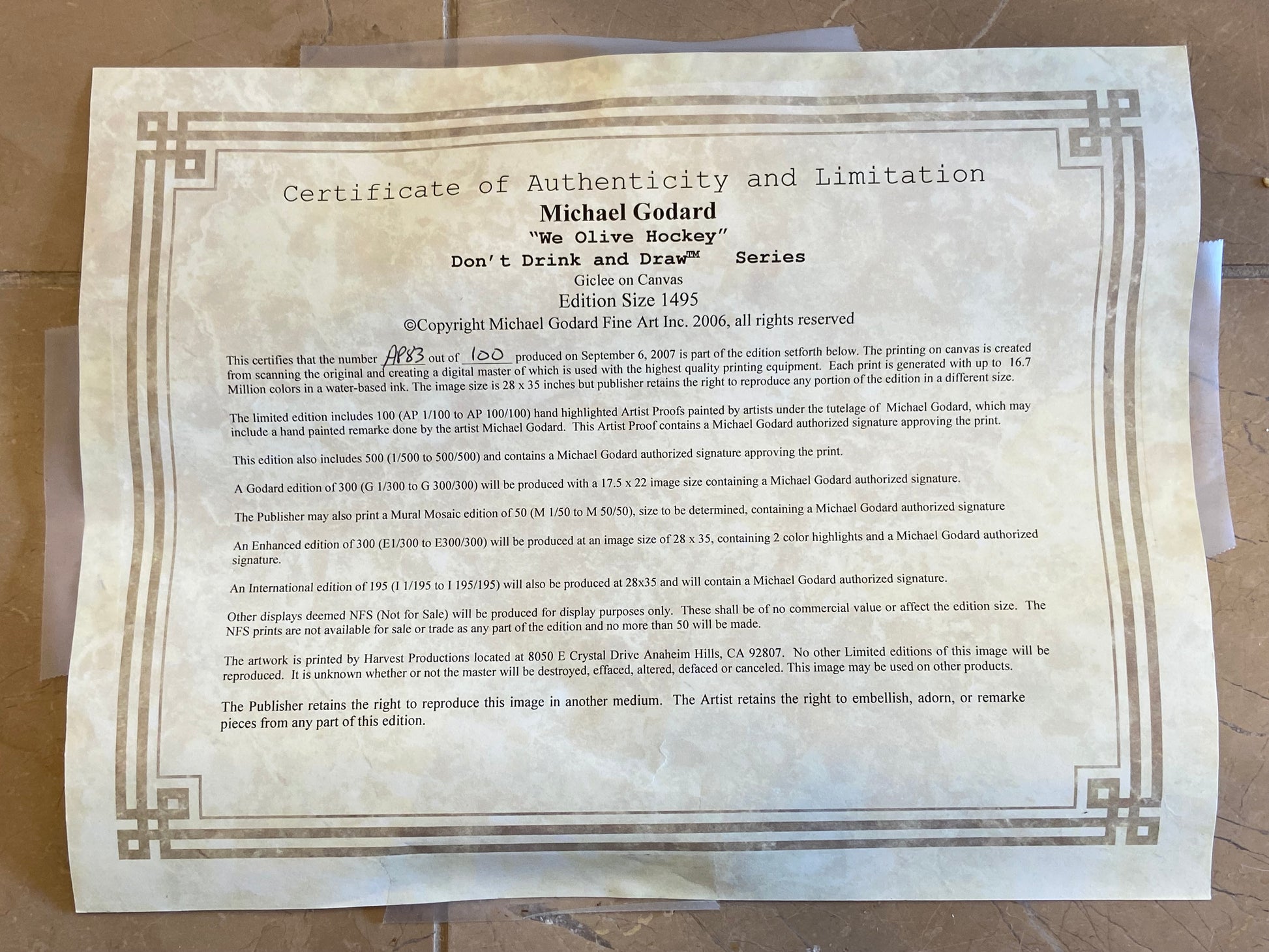The photograph, taken indoors, showcases a certificate that is taped to a light brown, stone-like wall with clear tape at all four corners. The certificate, displayed horizontally, features a parchment-style tan and cream-colored paper with a brown, marble-textured decorative border. The top of the certificate prominently reads "Certificate of Authenticity and Limitation" in bold lettering, followed by "Michael Goddard" and the phrase, in quotes, "We all live hockey." Below, it identifies the piece as part of the "Don't Drink and Draw Series" and mentions that it’s a "Giclee on Canvas Edition Size 1495," copyrighted in 2006 by Michael Goddard Fine Art Inc, with all rights reserved. Handwritten on the document is "AP 83 out of 100," indicating its unique number in the edition set. It was produced on September 6, 2007. The certificate goes on to detail the process and authenticity of the canvas prints, mentioning the use of high-quality printing equipment and the capability to reproduce up to 16.7 million colors. The rest of the certificate, packed with more details on the product and its authenticity, fills the bottom half of the paper.